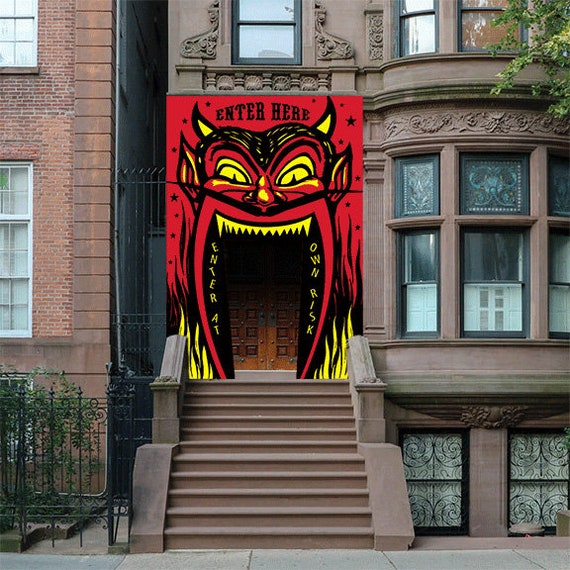This vivid, colored outdoor photograph captures a striking street-level view of an ornate, reddish-brown stone row home, likely from the 1800s, in a bustling metropolitan city such as New York or Detroit. The townhouse, appearing to have three stories, prominently features an eye-catching doorway. Approached by a set of steps from the sidewalk, the doorway is dramatically adorned with a painted panel resembling a gaping devil’s mouth, suggesting a seasonal or event-related decoration, perhaps for Halloween.

The devil's menacing face, with vibrant red coloring and black outlines, has yellow eyes, teeth, and horns, enhanced by yellow flames framing the mouth. Above the devil's mouth is a bold, black-lettered sign that reads "Enter Here," and on either side, warnings proclaim "Enter At Own Risk." The devil’s open mouth serves as a portal to the solid wood doors that lie behind it, accentuating the foreboding theme. Flanking the door are windows adding to the architectural charm of the home. The surrounding street scene is quiet, devoid of people, which further emphasizes the intriguing and slightly ominous focal point of the devilish entryway.